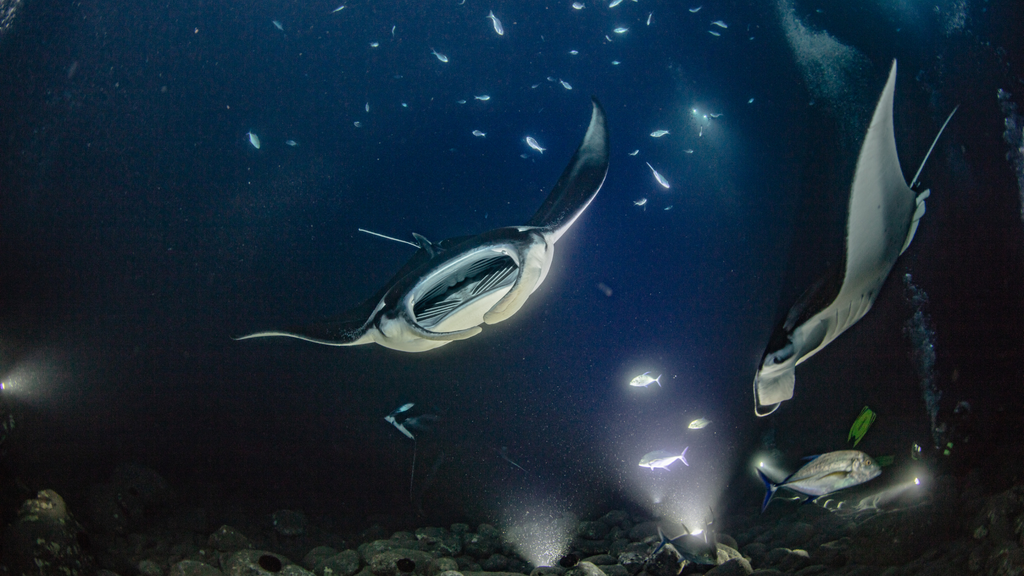This image captures a murky, predominantly dark aquarium scene viewed from outside the glass. The surrounding edges are intensely black, contrasting with the slightly illuminated center created by two lights at the bottom, casting a dim, darker blue hue. Scattered rocks cover the aquarium floor near these lights. Dominating the center is a head-on view of a large stingray, featuring a silver underside and a dark black top, its fins spread wide as it swims towards the camera. Swooping in from the top left corner, another stingray angles downward, displaying its silver underside and elevated tail. Toward the right side, a silver and blue fish swims toward another small light, while three smaller, white fish hover directly above it. The overall impression is of a murky, deep-sea environment, with varying sizes and types of aquatic life adding to the scene.